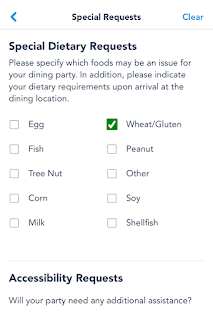A detailed screenshot of a food ordering app is displayed, specifically focusing on a section that allows users to customize their dietary requests. The top of the image features a bold heading that reads "Special Request" in black. Directly below this, another heading states "Special Dietary Request" followed by informative text that advises users to specify any foods that may cause issues for their dining party. Additionally, it instructs users to indicate their dietary requirements upon arrival at the dining location. The screenshot features two columns of checkboxes where users can mark their dietary restrictions. The left column lists: egg, fish, tree nut, corn, and milk. The right column lists: wheat, gluten, peanut, other, soy, and shellfish. This user-friendly interface aims to accommodate various dietary needs and preferences.